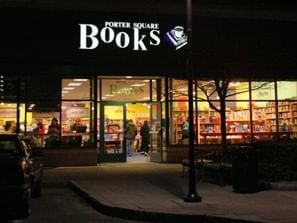This nighttime photograph captures the exterior of Porter Square Books, a brightly lit haven amidst the darkness. The store's top features bold white lettering spelling out its name against a black backdrop, flanked by an image of a black-and-white book topped with a coffee cup. The front is a showcase of expansive windows, divided by thin black strips, allowing clear views of the warmly illuminated interior. Inside, the yellow walls and numerous bookshelves are visible, along with a few patrons leisurely browsing. Outside the store, a barren tree and a tall light pole reach up to the top of the frame, enhancing the evening ambiance. The sidewalk in front features a half-visible parked car on the left side, a bench, and a trash bin. On the right side, a small bush adds a touch of greenery to the scene.